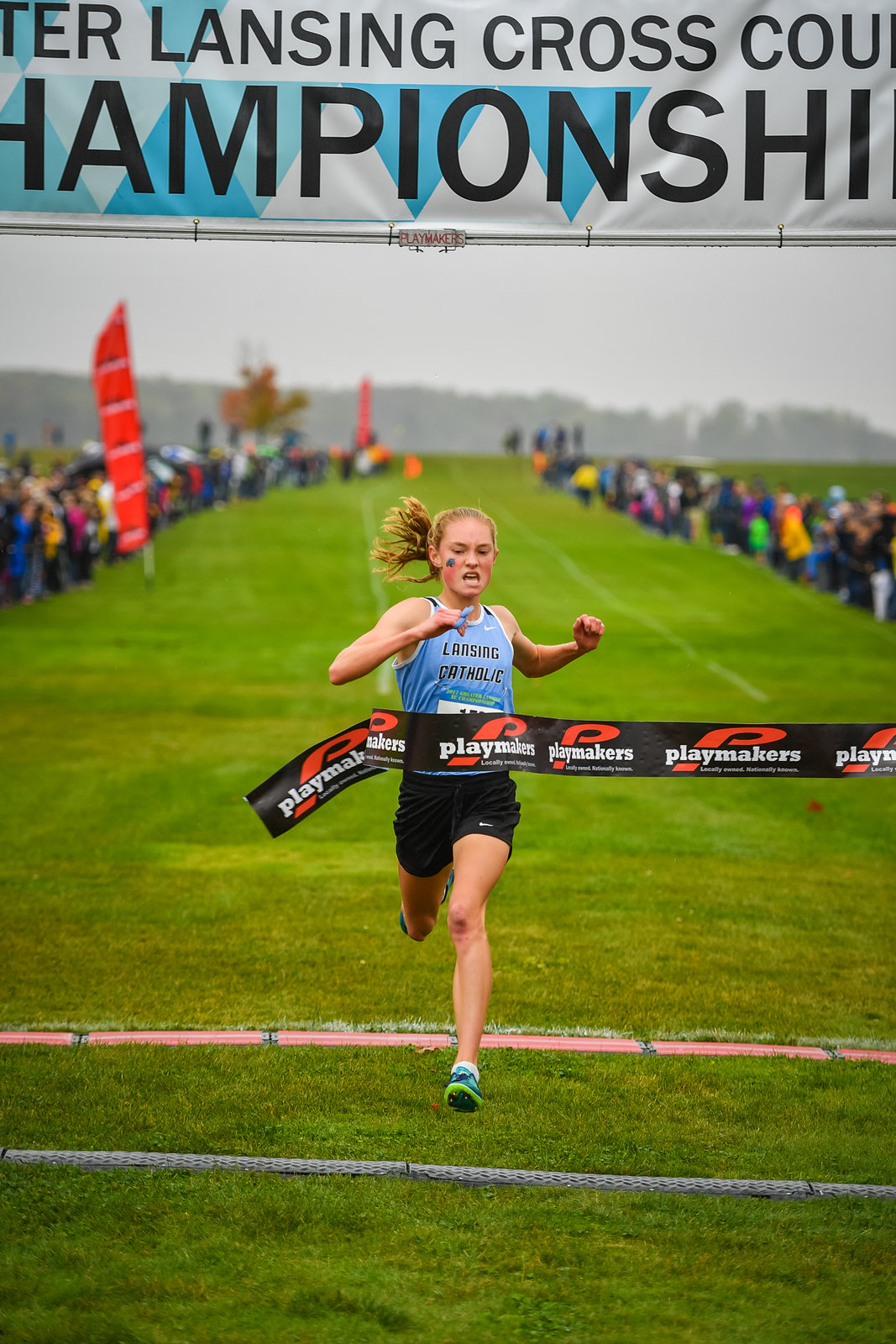The photograph captures the decisive moment of a cross-country race at the Greater Lansing Cross-Country Championship. A determined girl, wearing a blue tank top with "Lansing Catholic" written on it and black shorts, sprints across a pristine green field, breaking through a finish line banner that reads "Playmakers" in white against a blue background. Her face displays a mix of exhaustion and determination, with her hair pulled back in a ponytail and a distinct mark of makeup on her right cheek. Spectators line both sides of the field, creating an empty central lane for the runners. Behind her, there are two red flags held by people on her left, and an overcast sky with a row of leafy trees in the background completes the backdrop. She clutches something blue in her right hand and wears blue and green shoes, crossing orange markers and a chalk-drawn blue line as she finishes the race alone, with no other runners in sight.